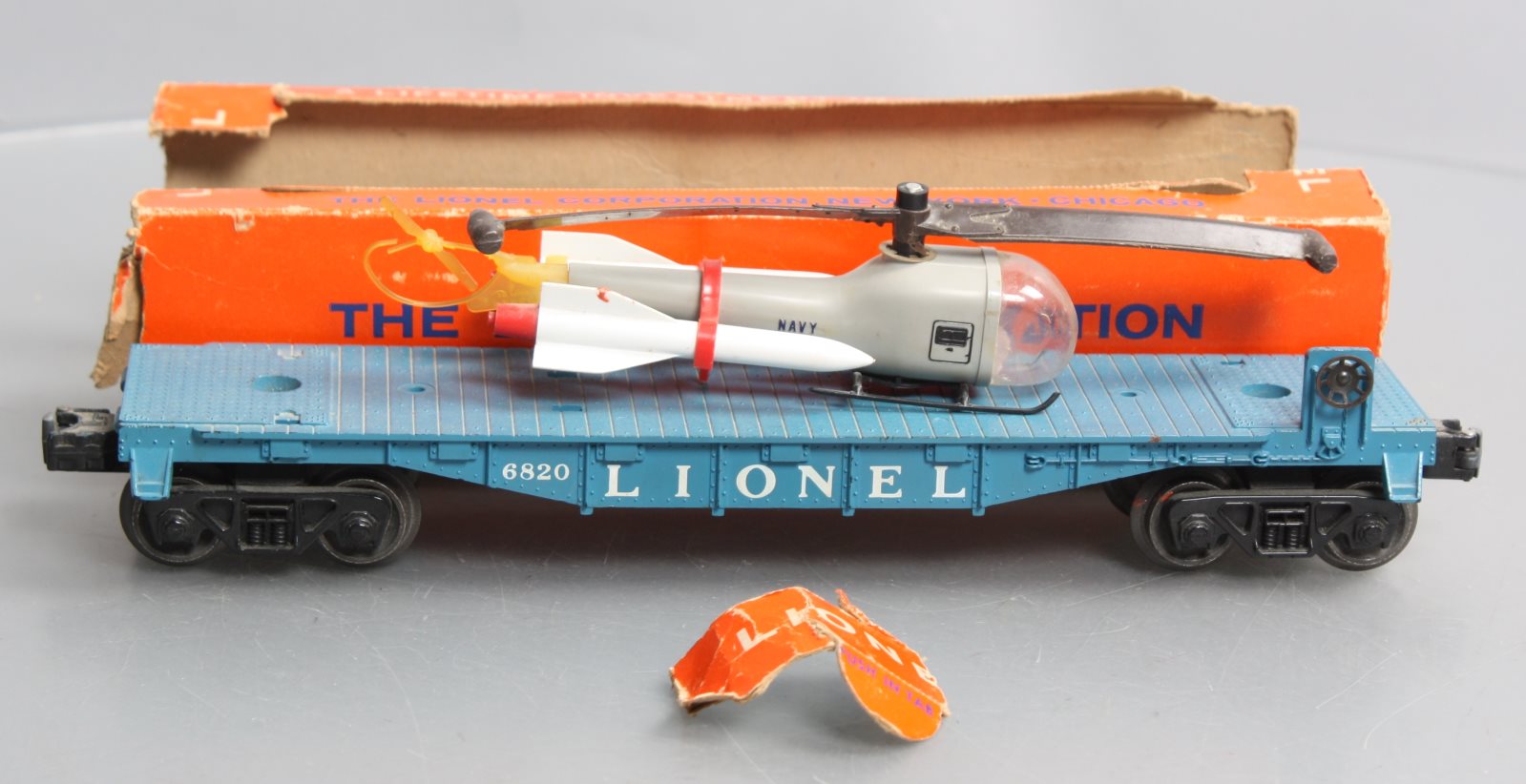This rectangular image, about twice as wide as it is tall, features a detailed scene set against a light gray background with a subtle curved groove at the top. Central to the image is a medium blue flatbed train car labeled "Lionel" in white letters, accompanied by the number "6820". Atop the flatbed sits a detailed white and gray helicopter, affixed with a small red tie and a white object resembling a missile or a golf tee. Behind the flatbed train car is an antique, orange cardboard box with some portions of text visible, suggesting age and wear. The box, clearly associated with the Lionel brand, has a torn piece placed in front of the flatbed, emblazoned with the letters "L-I-O-N." The entire arrangement is situated on a light gray surface, contributing to the image's nostalgic and vintage feel.